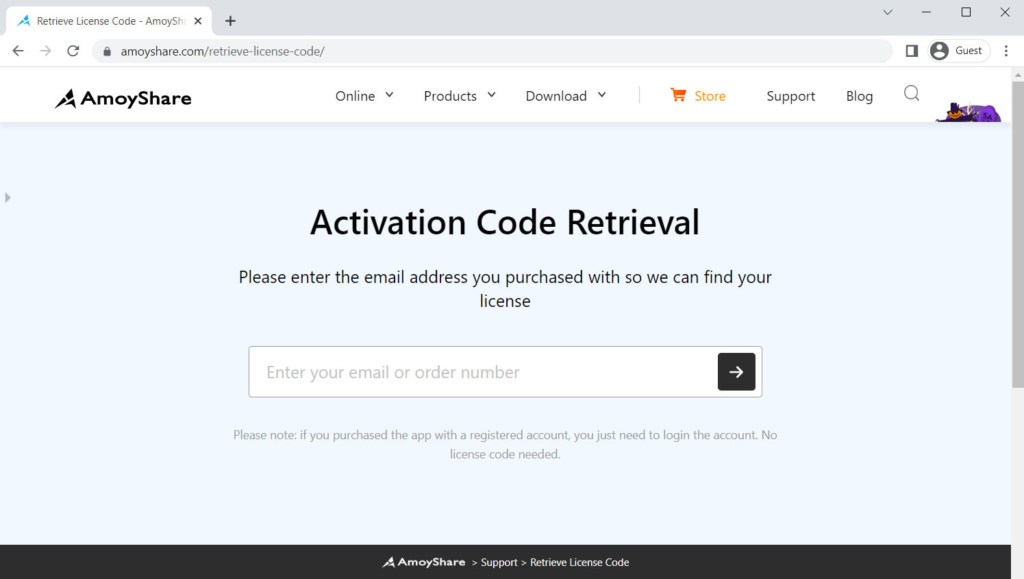In this image, we see a screenshot of a web page displayed on a mobile device, specifically focusing on a tab that is open to the "Retrieve License Code" section of the Amoishare website. The URL in the address bar reads "https://www.amoishare.com/retrieve-license-code/". The navigation bar at the top includes several links: "Online", "Products", "Download", "Store", "Support", "Blog", and a search icon. The main content of the webpage features a header titled "Activation Code Retriever" followed by a prompt instructing users to enter the email address used at the time of purchase to retrieve their license code. The placeholder text in the input field suggests users can enter their "email or order number". Additionally, there is a note explaining that if the app was purchased with a registered account, logging into that account would suffice, and no license code would be needed. At the bottom of the page, there are links for "Amoishare Support" and "Retrieve License Code". The clean layout and clear instructions are designed to facilitate easy license code retrieval for users.